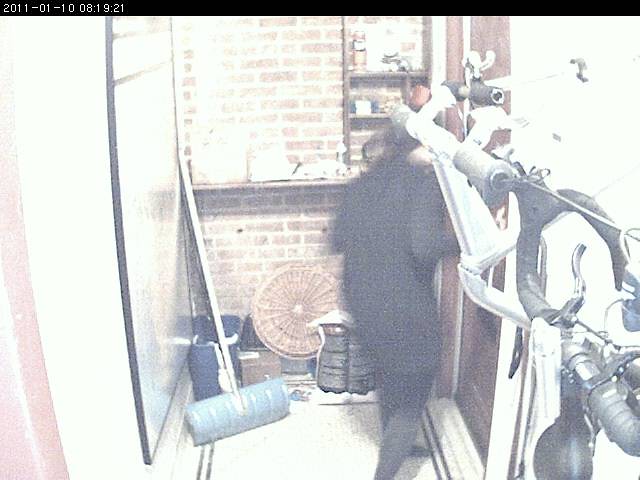A grainy and slightly blurry black-and-white image seemingly captured by a security camera. The top-left corner of the image features a black banner with white text displaying the date "2011-01-10" and the time "08:19:21." The scene takes place inside some kind of store, where a person can be spotted. The background includes a brick wall adorned with various items, one of which appears to be a shovel. Despite the image's low resolution, the individual seems to be looking through a window or similar structure.